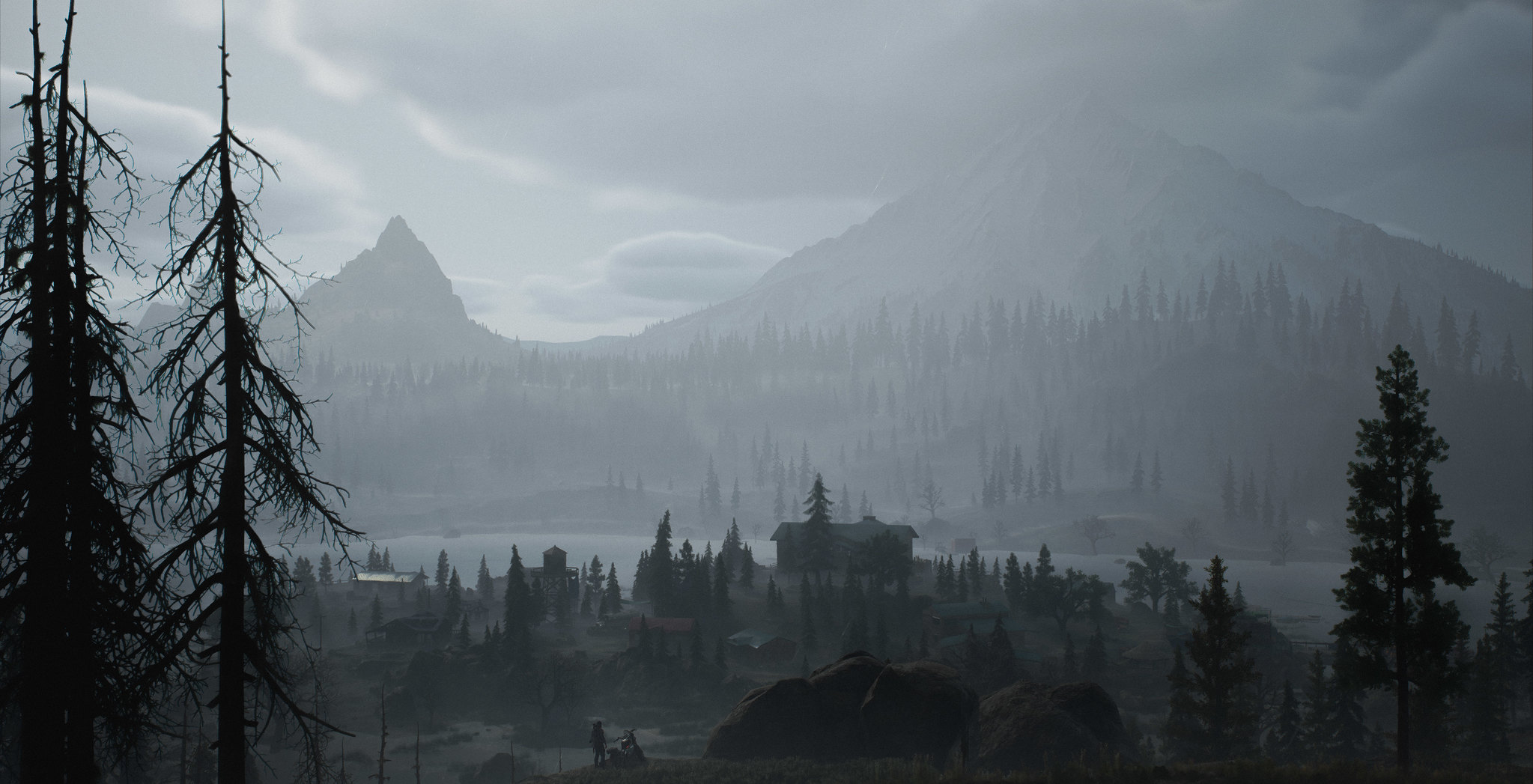This landscape image, potentially a photograph or a computer-generated rendering, captures a serene and picturesque scene. In the far background, towering mountains with snow-capped peaks blend into a sky dotted with fluffy clouds. Moving toward the middle of the image, a dense forest of lush trees stretches across the landscape, leading to a gently flowing river. Along the riverside, scattered structures that appear to be houses add a touch of human presence to the natural environment. In the very foreground, the scene is framed by trees on both the left and right sides, flanking the view. Large boulders are strewn across this front area, and a couple of diminutive figures, likely people, can be seen, adding a sense of scale to the expansive scenery.